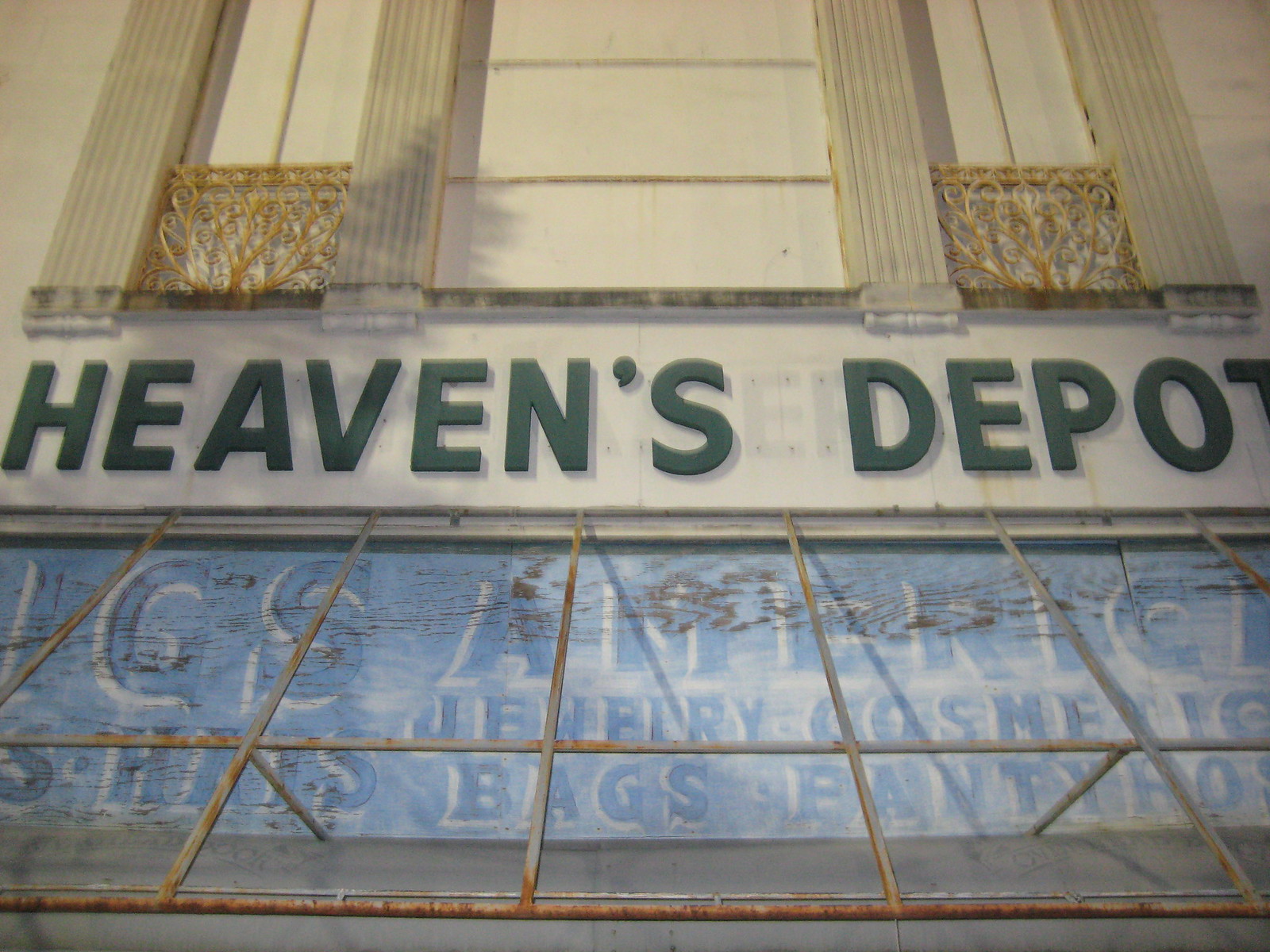This image captures a detailed view of a building featuring a prominent sign that reads "Heaven's Depot" in green letters. The sign is mounted on a tan rectangular background, seamlessly integrated into the architectural design of the building. Flanking the sign are tan pillars, which support intricate golden gates nestled between them. Below the sign, portions of the building's façade include glass panels that are partially obscured by metal poles; the text on these glass sections is blurred and undecipherable. The overall aesthetic of the structure blends modern and classical elements, highlighting the "Heaven's Depot" signage as a focal point.